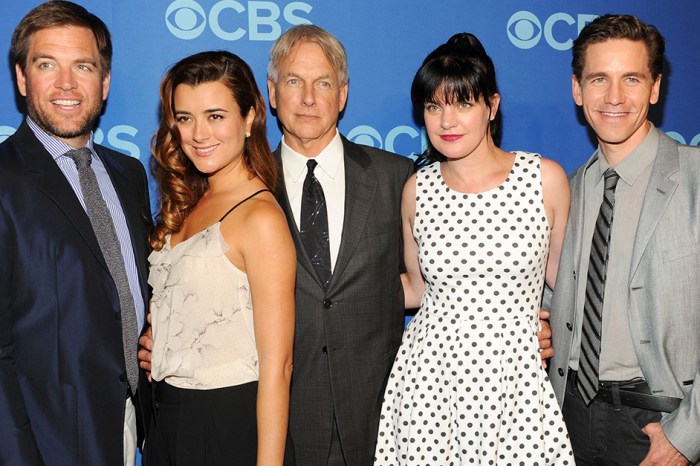This image showcases five cast members from the television show NCIS, standing in front of a solid blue backdrop adorned with the CBS logo in light blue. Front and center is Mark Harmon, immediately recognizable, dressed in a classic dark suit and tie. To his right is a female lead in a white dress adorned with black polka dots, her dark hair styled down. Next to her stands a male actor in a black suit jacket and speckled tie, with a white collared shirt, sporting a clean-shaven look. On Mark Harmon's left, another leading actress wears a sleeveless, ruffled white blouse paired with black bottoms, her hair elegantly curled. Completing the group is a man to her left in a navy blue suit jacket, gray tie, and light blue collared shirt, smiling as he gazes into the distance. The clean and professional attire, alongside the CBS logo backdrop, emphasizes the formal and polished nature of the event.